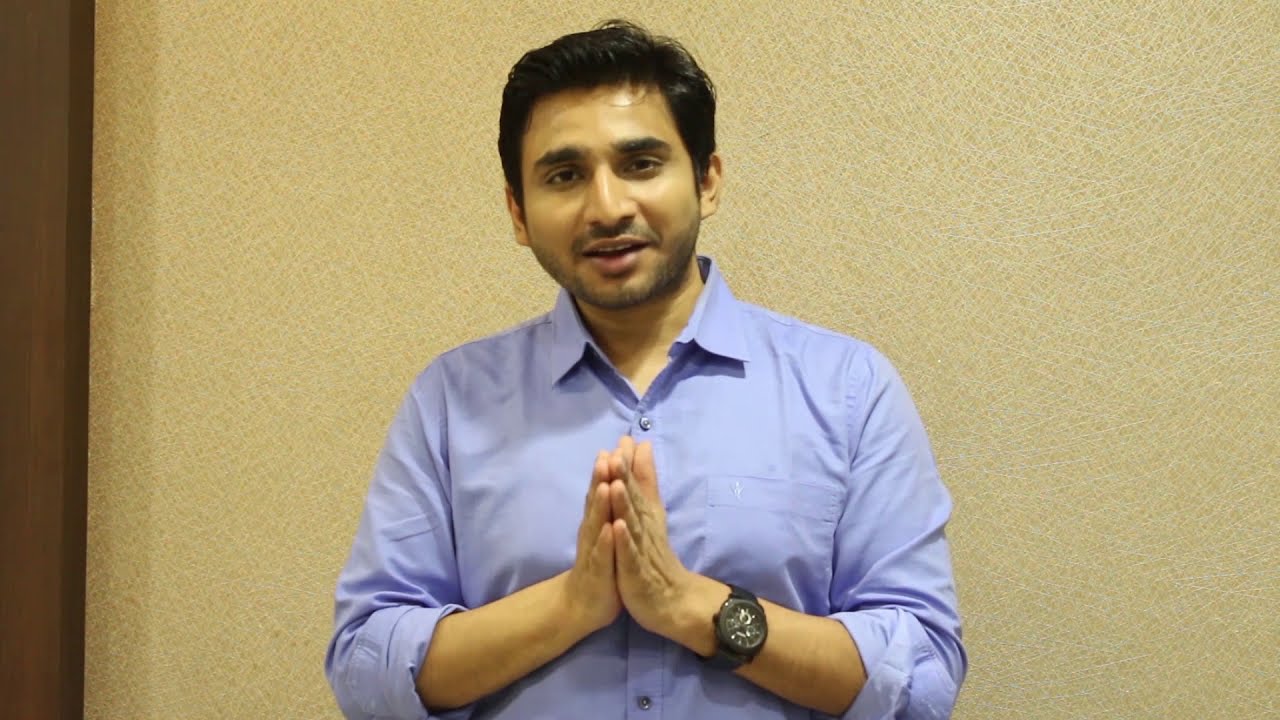The photograph features a man standing inside a building against a cream-colored wall with some light patterning. To the man's right, the wall has a black-brown trim that suggests the edge of a doorway. The man is facing the viewer directly, appearing to be in mid-speech with his mouth slightly open, revealing the top row of his teeth. He has short black hair and sports a light 5 o'clock shadow beard and mustache. His skin tone is a lighter brown, and he has dark eyebrows and brown eyes. He is dressed in a long-sleeved, baby blue button-down shirt with the sleeves rolled up to his forearms. On his left wrist, he wears a large black watch. The image captures him from the waist up, with his hands pressed together in front of him in a prayer-like fashion, fingers pointing towards the camera.